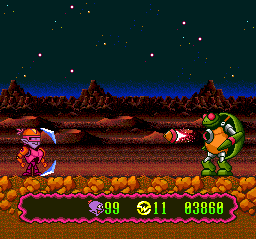This image captures an intense moment in a retro-style computer game, featuring a science fiction battle scene. In the foreground, two distinctive figures are locked in combat. On the right stands a formidable, armored turtle-like creature with red eyes, launching a rocket from its chest. This character, resembling a blend of classic Ninja Turtle aesthetics and futuristic design, has a vivid green shell. Opposite it, on the left, is a smaller, purple elf-like figure with pointed ears, dressed in striking pink and orange armor, and holding a stylized shield in defense. The backdrop sets a desolate, extraterrestrial stage with barren hills and mountains that fade into a royal blue horizon beneath a star-studded night sky. Across the bottom of the screen, the game's score display reads '99' for the purple elf, '11' associated with a 'W' in an orange circle likely representing the turtle, and an enigmatic '03860'.